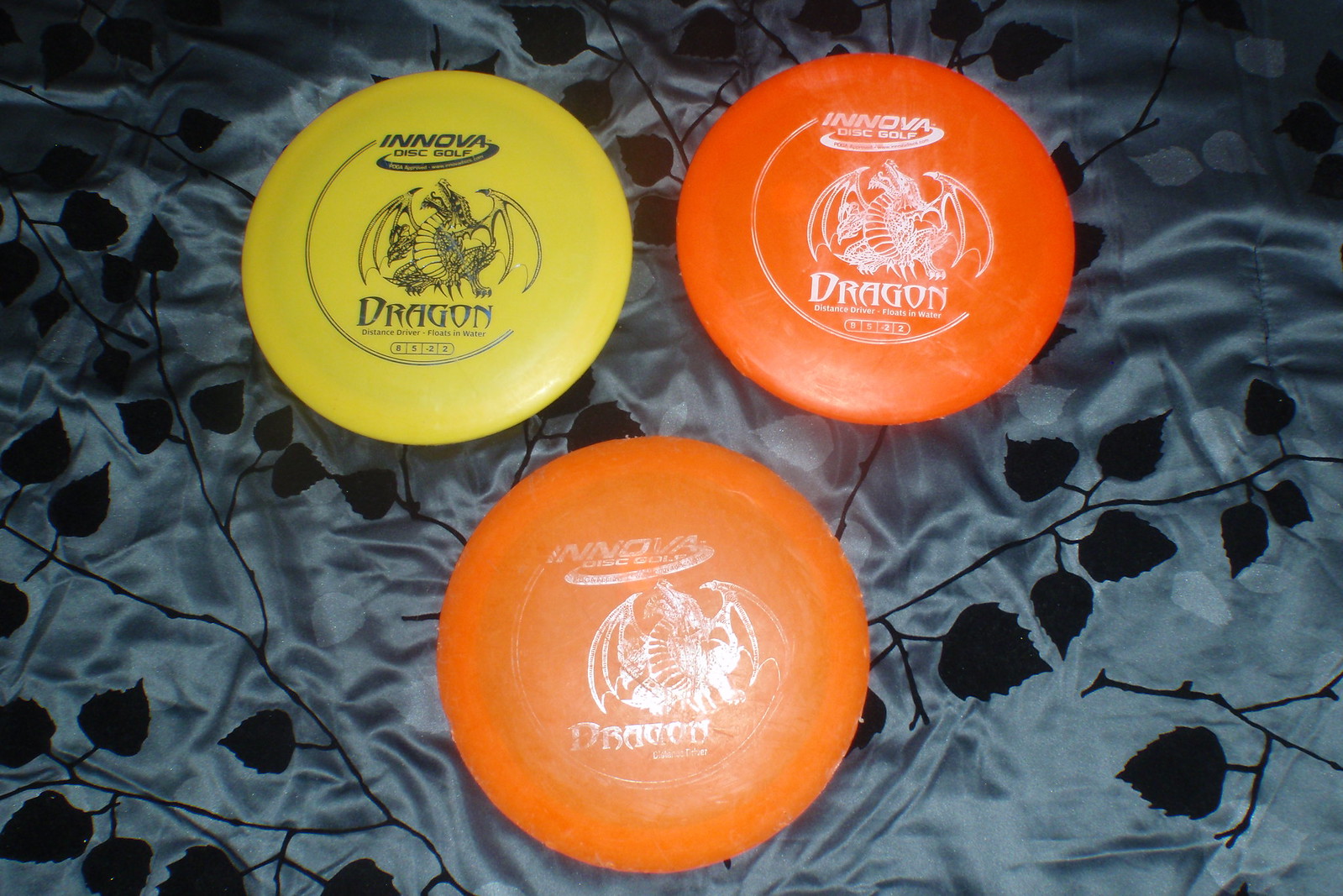This image features three disc golf discs laid out in an upside-down triangle formation on a slate blue comforter with a black leaf and branch pattern. The discs, manufactured by Innova Disc Golf, each prominently display a fine-line logo of a dragon with text reading "Dragon Distance Driver" and "Floats in Water." The top left disc is bright yellow with black ink for the logo and text. The other two discs are shades of orange: the top right one is a more vibrant orange with a silvery logo, while the bottom disc is a lighter, more faded orange, indicating heavier use. The intricate design of the dragon on each disc shows it with its mouth open, wings spread, and looking upwards, with a circular line extending from the Innova logo around the dragon. The photograph is taken from a top-down perspective, with lighting that creates a slight reflection on the discs, suggesting the use of a flash.